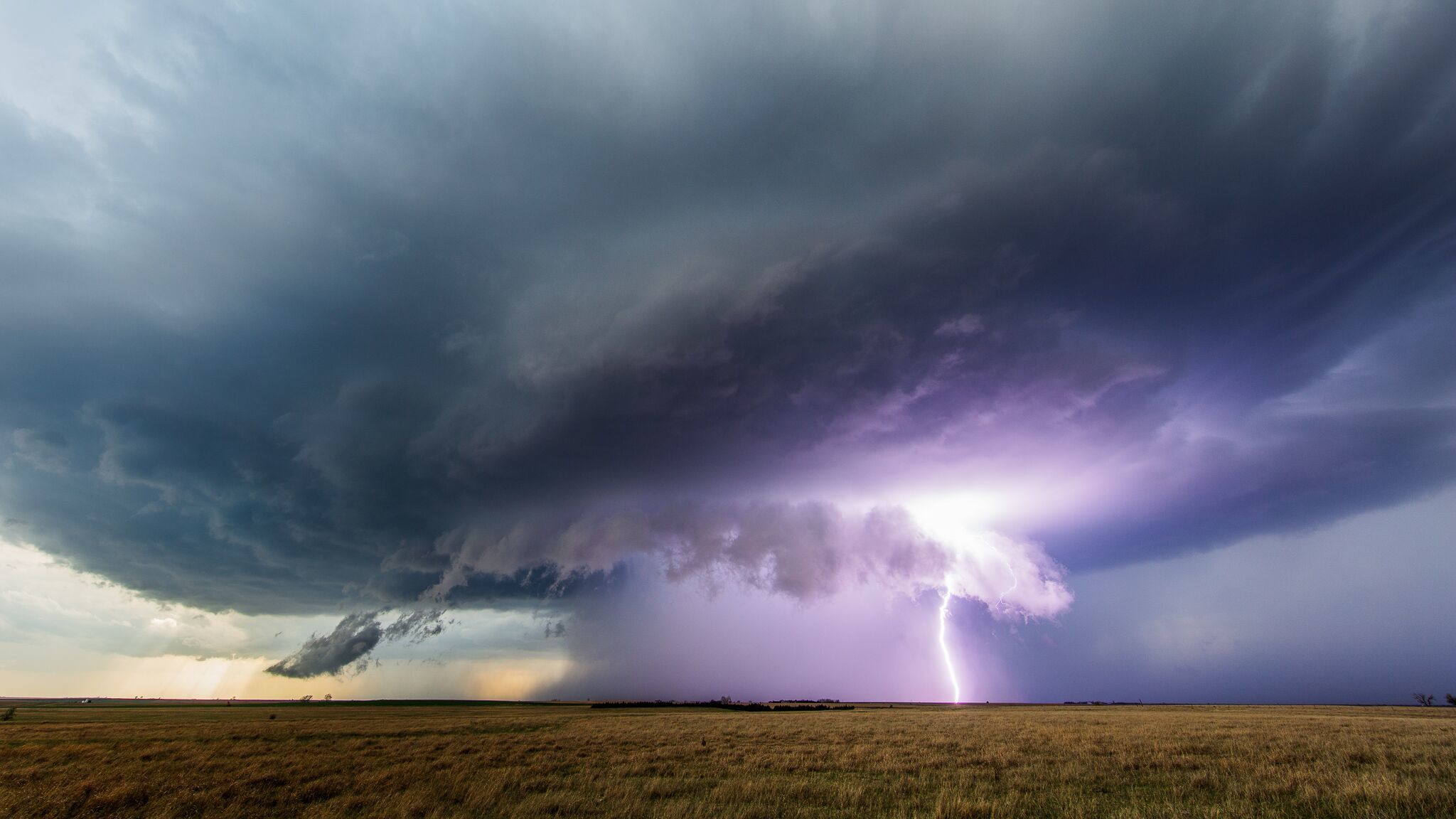This landscape photograph captures a striking storm over an expansive field, dominated by a tumultuous sky. The image, horizontally aligned, features a small strip of golden-brown grassland or farmland occupying the bottom sixth of the frame, highlighted by a flat horizon without any hills. Above, dark, imposing storm clouds fill the sky, creating a dramatic and ominous atmosphere. 

In the center of the image, a column of rain descends from the cloud cover to the ground, surrounded by the round, underbelly of the storm cloud. This section of the sky is illuminated in a light lavender hue, intensifying the visual impact of the scene. Approximately three-fifths of the way to the right of the image, a brilliant lightning bolt strikes the ground, casting a stark, glowing light that further enhances the purple and white hues in this area.

The immense supercell presents a powerful display of nature’s force, with the dynamic colors and textures of the clouds and lightning creating an awe-inspiring spectacle over the open plain. The vastness of the terrain, with only a few distant trees visible, emphasizes the sheer scale and intensity of the storm, making this an unforgettable depiction of a formidable weather event on the Great Plains.